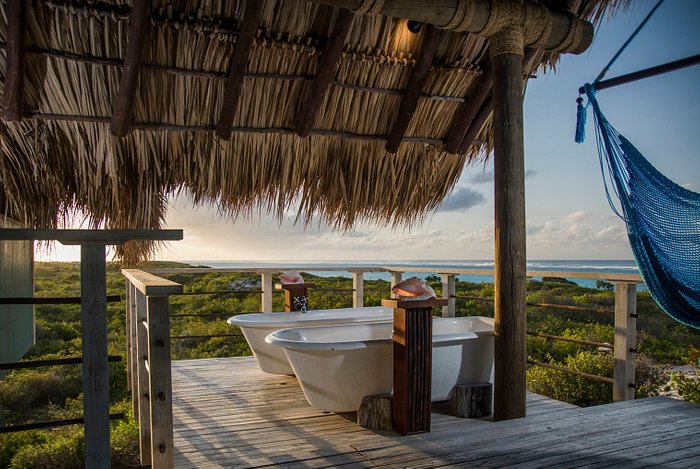The image depicts a picturesque scene of a balcony at a tropical resort. The balcony is made of sturdy, unfinished wooden planks, supporting two large white porcelain bathtubs. Adjacent to the tubs stands a monolith-like structure, likely a water feature that fills the tubs. To the right, a blue hammock chair hangs, adding a touch of relaxation to the setting. A thatched roof made of dried grass and wood provides an idyllic, rustic awning. The balcony offers an elevated view of lush greenery and shrubbery, stretching out to reveal the brilliant blue of the ocean in the distance. The sky, adorned with some clouds, suggests it is either sunrise or sunset, casting a serene and warm light over the entire scene.